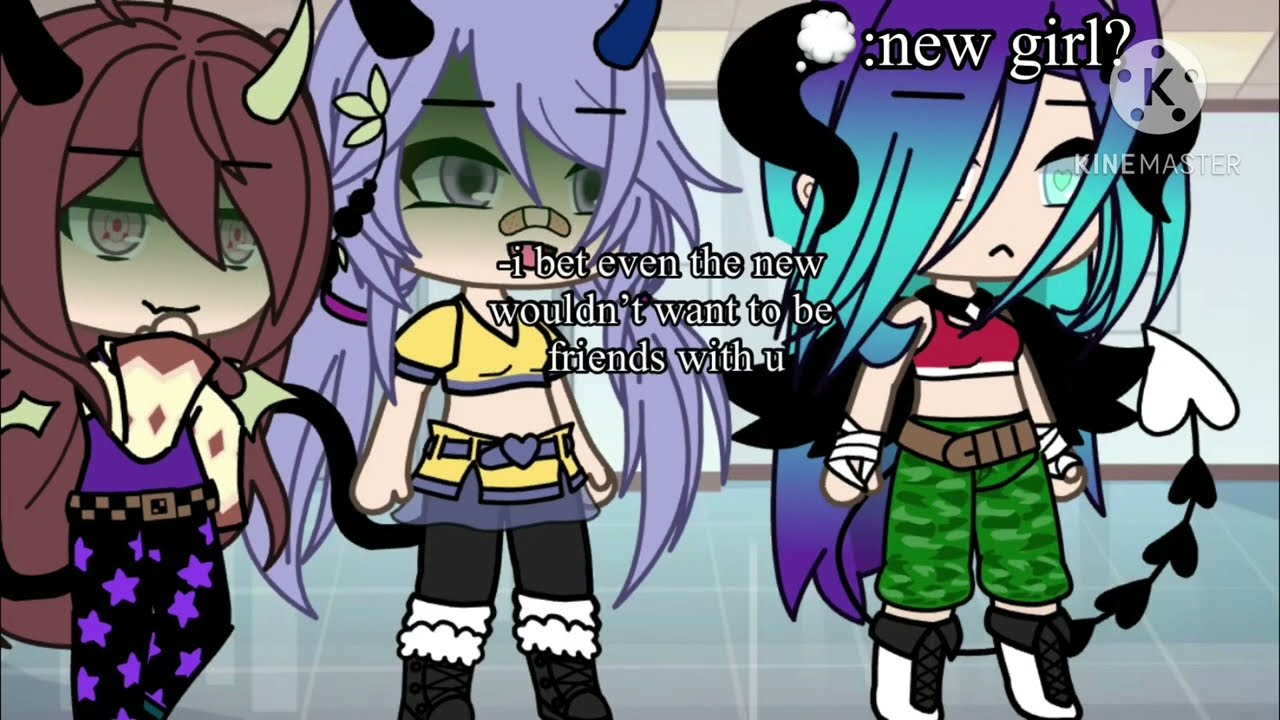In a scene reminiscent of a Japanese-style cartoon or video game still frame, three distinct cartoon girls with small horns stand side-by-side on a light blue floor against a white wall with a low beige ceiling. The girl on the left has long brown hair, adorned with a black horn on the left and a yellow horn on the right side of her forehead. She wears a purple outfit cinched with a brown belt and pairs it with black pants decorated with purple stars. The middle girl, featuring long light purple hair, sports a yellow outfit with black pants and boots, and has a black horn on the left and a blue horn on the right of her forehead, with a small band-aid on her nose. The girl on the right has long hair colored in purple and green and is dressed in a red top, green pants, and red boots. Across the middle of the image, a bold white text outlined in black reads, "I bet even the liu wouldn't want to be friends with you," suggesting a scene of confrontation. The top of the image includes a logo with a 'K' and text questioning "new girl?" hinting at the introduction of a new character or element in the scene.